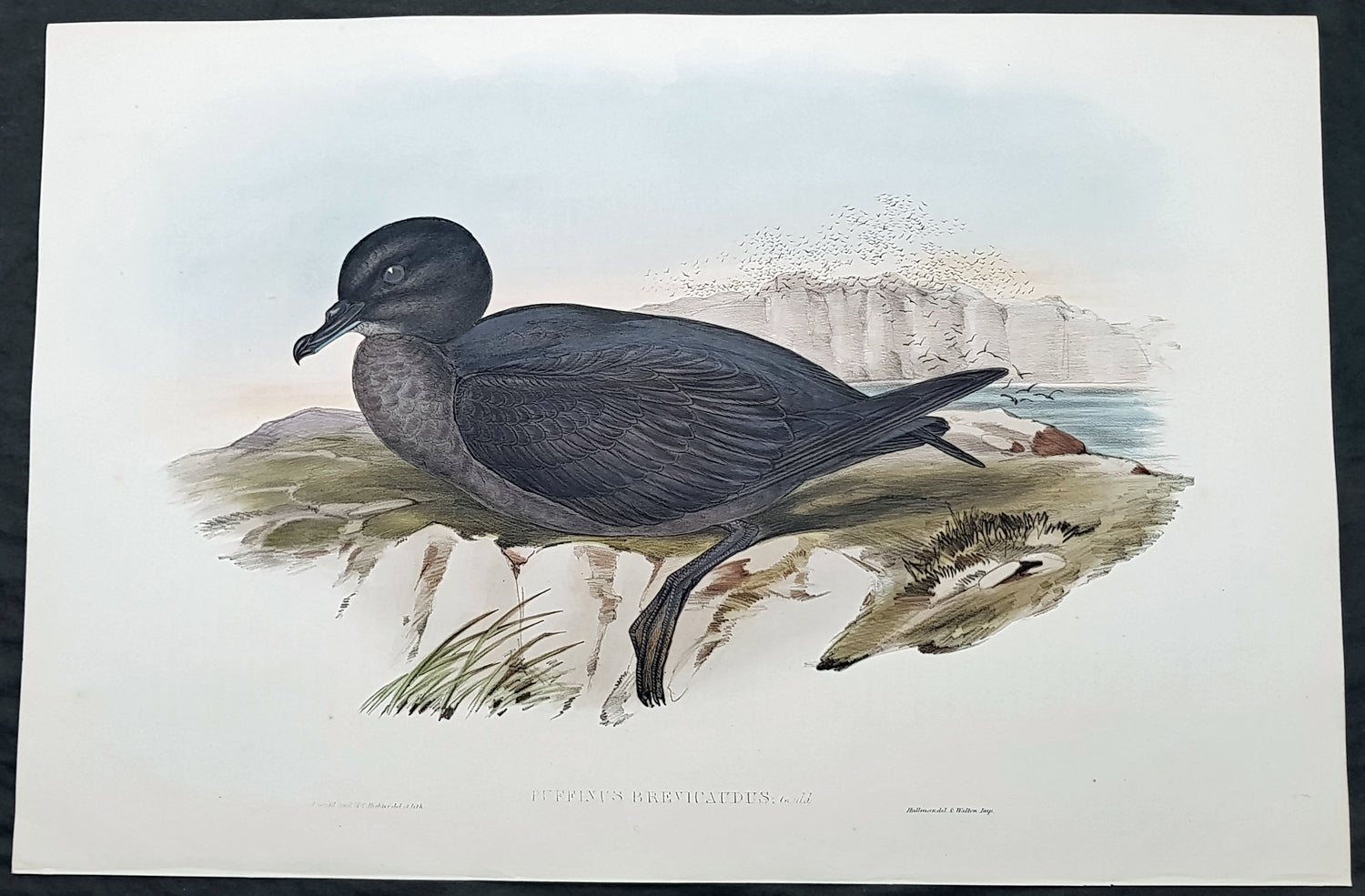This image features a watercolor painting of a bird. The background is predominantly white with subtle elements, including a pale blue sky at the top center and a light gray mountain range faintly visible beneath it. Below the mountain, a few light brush strokes suggest a body of water, potentially a lake or stream. The scene is painted in delicate, pastel tones.

In the foreground, the bird is depicted in a side profile, perched on a rocky ground that has patches of flat green and some sparse sea grasses. The bird itself has a dark gray, almost bluish black plumage, with a speckled slate gray breast highlighted by darker spots. It has a small, intense-looking beak that is black and slightly curved at the end, as well as black feet and a single visible black eye.

The painting beautifully captures the essence of the bird and its simple, yet evocative surroundings with minimalistic and soft watercolor strokes.